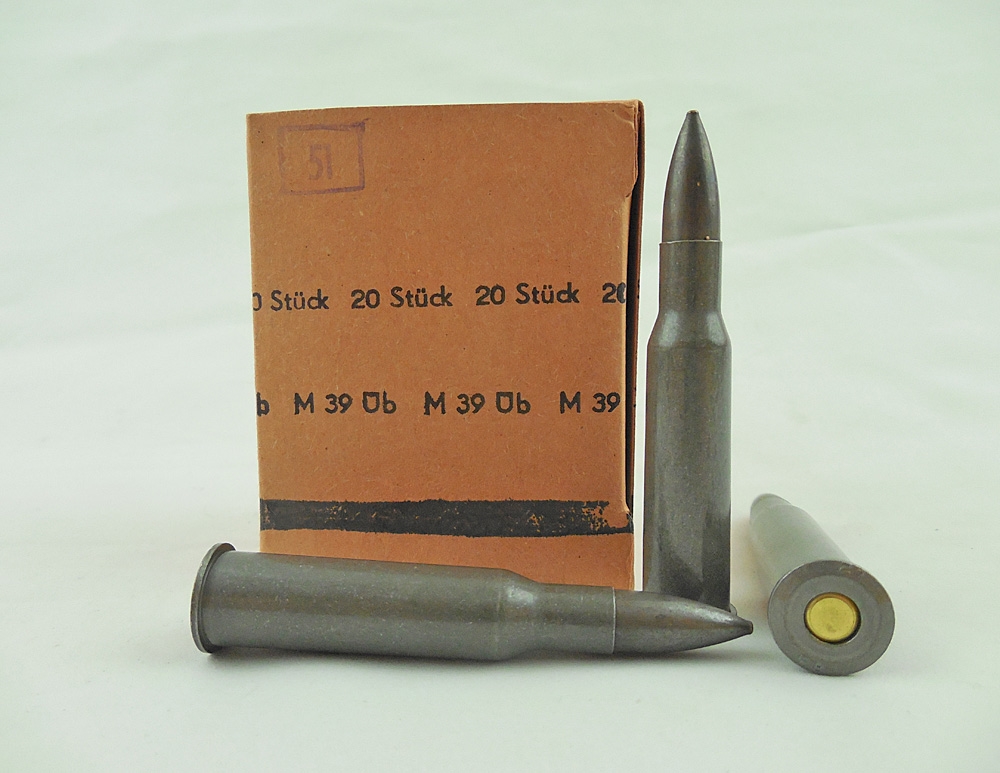The photograph showcases three bullets arranged on a lime green surface, which appears smooth, possibly indicative of either a table or a studio setup. One silver bullet lies horizontally on the ground with its tip pointing towards the right. To its right, another bullet lies horizontal but reversed, displaying its base with a small yellow material visible in the center. The third bullet stands vertically on its base, pointing upwards, near a brown folded cardboard piece about the same height as the standing bullet. The brown cardboard shows a pattern repeated across it with the text "STÜCK 20," "M39," and images of a shield followed by the letter "B." The bullets themselves have a dark, brownish-green hue.